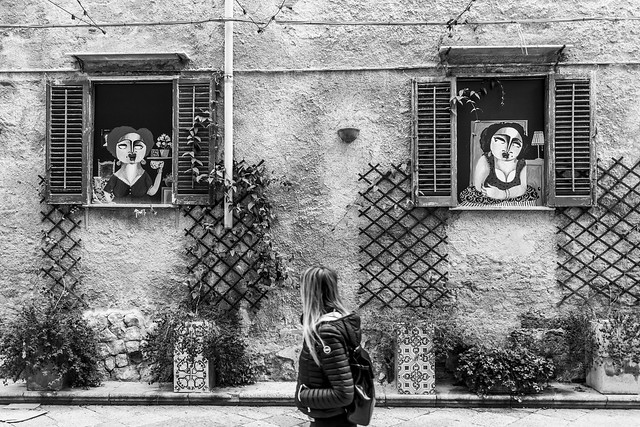In this black and white photograph, a young woman with long hair, possibly blonde, is seen from the side as she walks down a street, her face turned away from the viewer. She is wearing a long, dark coat with her hand in the pocket and has a backpack on her back. The woman's attentive gaze is fixed on the building to her right, which features two windows with shutters. Each window displays an abstract or cartoon-like image of a woman. In the left window, the woman is holding a tray with a flower, and a dining room table with one chair is visible behind her. The woman in the right window is dressed in a gown, and behind her is a doorway and a nightstand with a lamp. Both figures appear to be looking outwards towards the street. The building, possibly reminiscent of Mexican or Italian architecture, has a stone or stucco facade with crosshatched lattices for vines, adding a touch of greenery. Below the windows, there is grass or bushes lining the clean sidewalk, suggesting it is daytime in this serene urban setting.